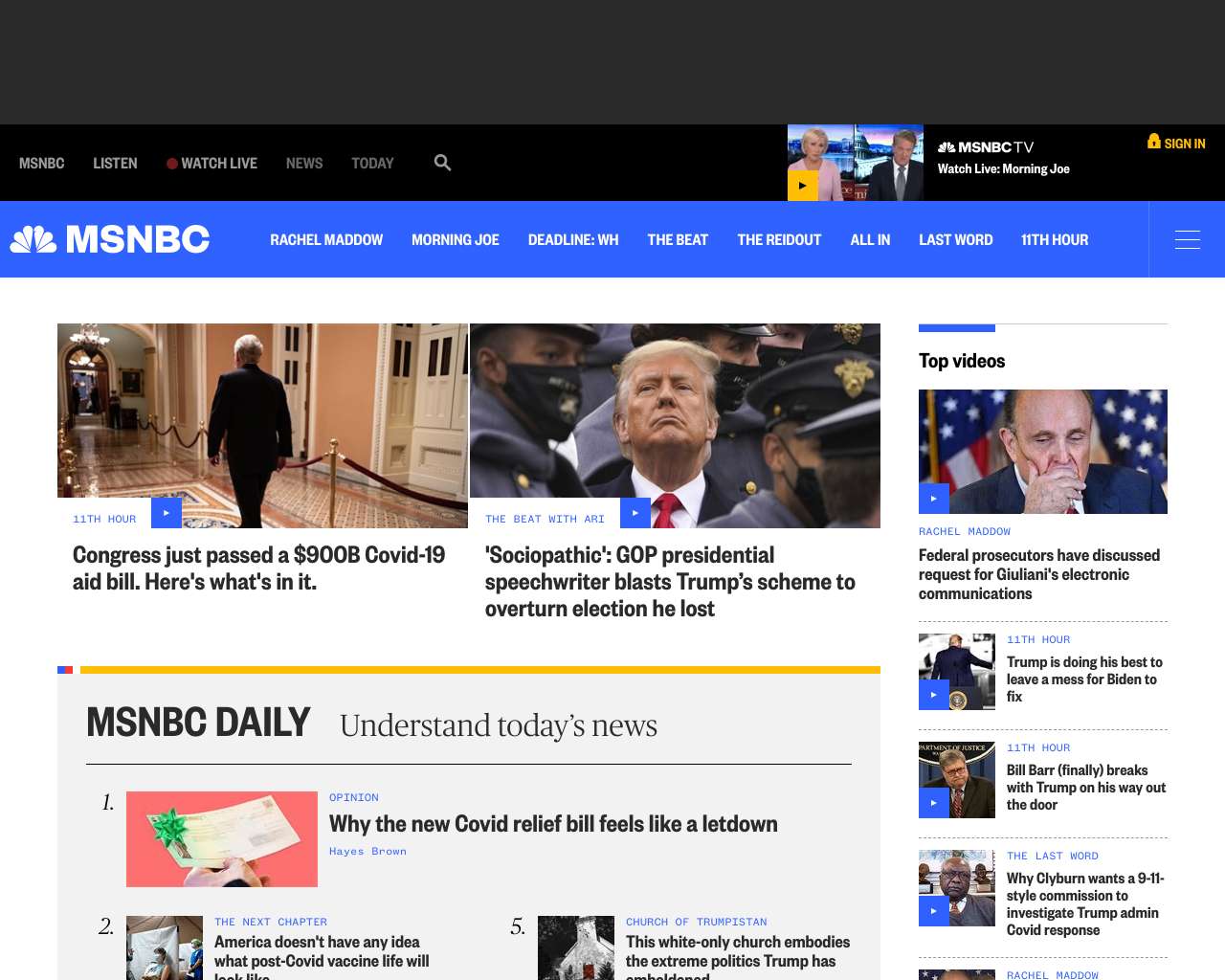Screenshot of MSNBC Web Page:

The screenshot captures the MSNBC web page in detail. At the top of the page, a video box features Morning Joe and Mika with an option to watch Morning Joe live on MSNBC TV. A sign-in button is prominently situated on the right. To the left of the video box, various options are arranged, including MSNBC, Listen, Watch Live, News, Today, and a search bar. Below this, a horizontal blue banner spans the width of the page, adorned with the NBC logo on the left and flanked by options like MSNBC, Rachel Maddow, Morning Joe, Deadline, White House, The Beat, The Readout, All In, Last Word, and 11th Hour on the right.

The section beneath the blue banner features a white background with a series of stories listed. Key headlines include "Congress Passes $900 Billion COVID-19 Aid Bill, Here's What's In It" and "Sociopathic GOP Presidential Speechwriter Blasts Trump's Scheme to Overturn Election He Lost." To the right, running vertically down the page, a series of video segments are highlighted with titles such as "Federal Prosecutors Discuss Request for Giuliani's Electronic Communications," "Trump Is Doing His Best to Leave a Mess for Biden to Fix," "Bill Barr Finally Breaks with Trump on His Way Out the Door," and "Why Clyburn Wants a 9/11 Style Commission to Investigate Trump Admin COVID Response."